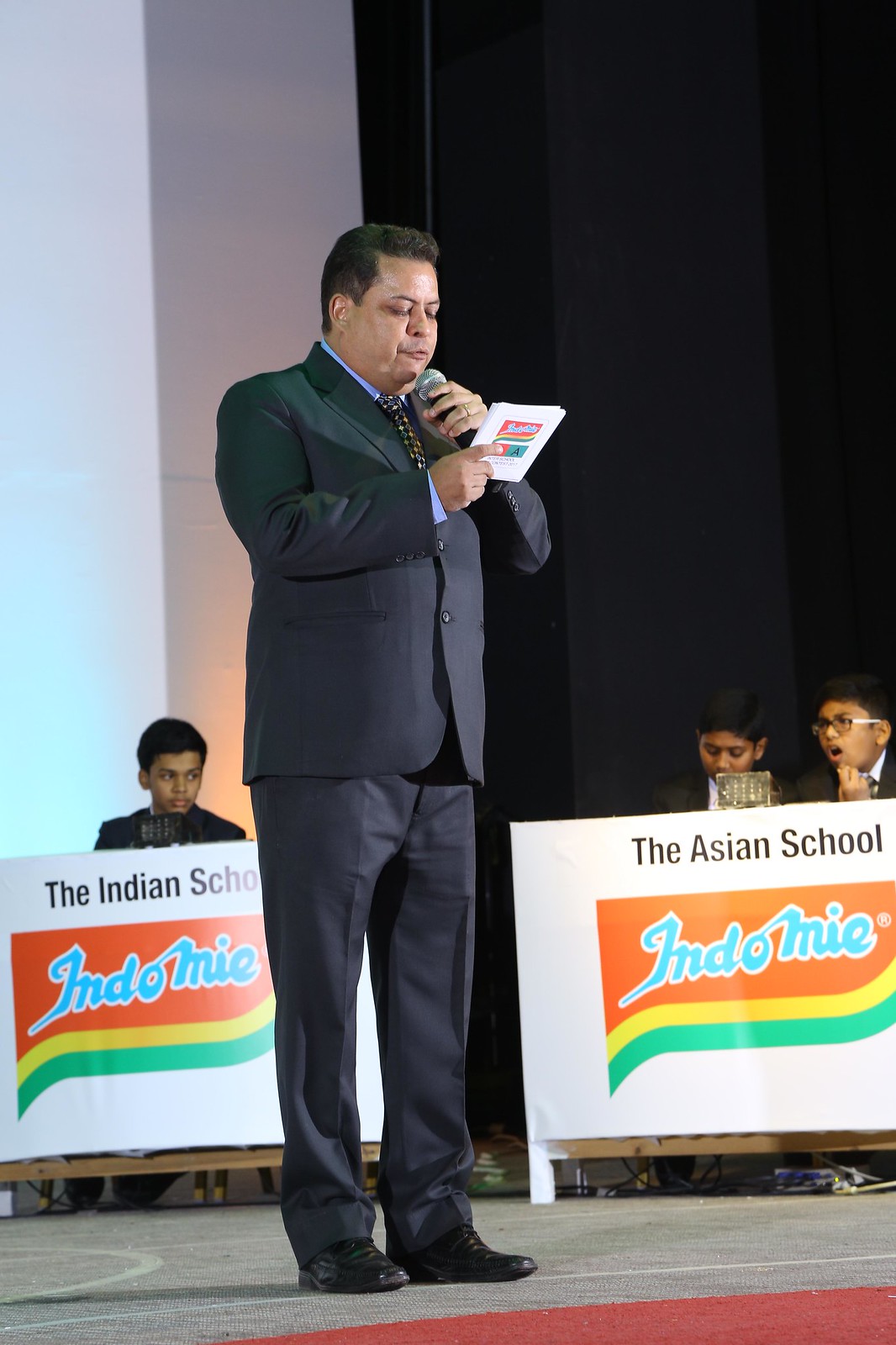The image depicts a man of likely Indian descent standing on a stage, delivering a speech into a microphone while holding a stack of index cards. He is dressed in a buttoned-up black business suit with a light blue collared shirt and a tie with specks, complemented by well-pressed black pants and shiny black shoes. He stands on a light brown carpet with a hint of red. The background features a juxtaposition of a white wall to the left and a dark black curtain to the right.

In front of him, there are tables behind which sit neatly dressed individuals, appearing to be South Asian students around the age of 13. Some are dressed in suits or collared shirts, and at least one wears glasses. They are seated behind large signs that read "The Asian School Indomie," with the logo displaying waves in orange, yellow, and green. This logo is also present on the index cards the man is holding, indicating that the event may be connected to the school or part of a game or quiz. Bottles of water are placed on the tables. The students' attire suggests they might be in uniform, and they appear to be engaged in the proceedings, possibly involved in a trivia game as suggested by the setup.